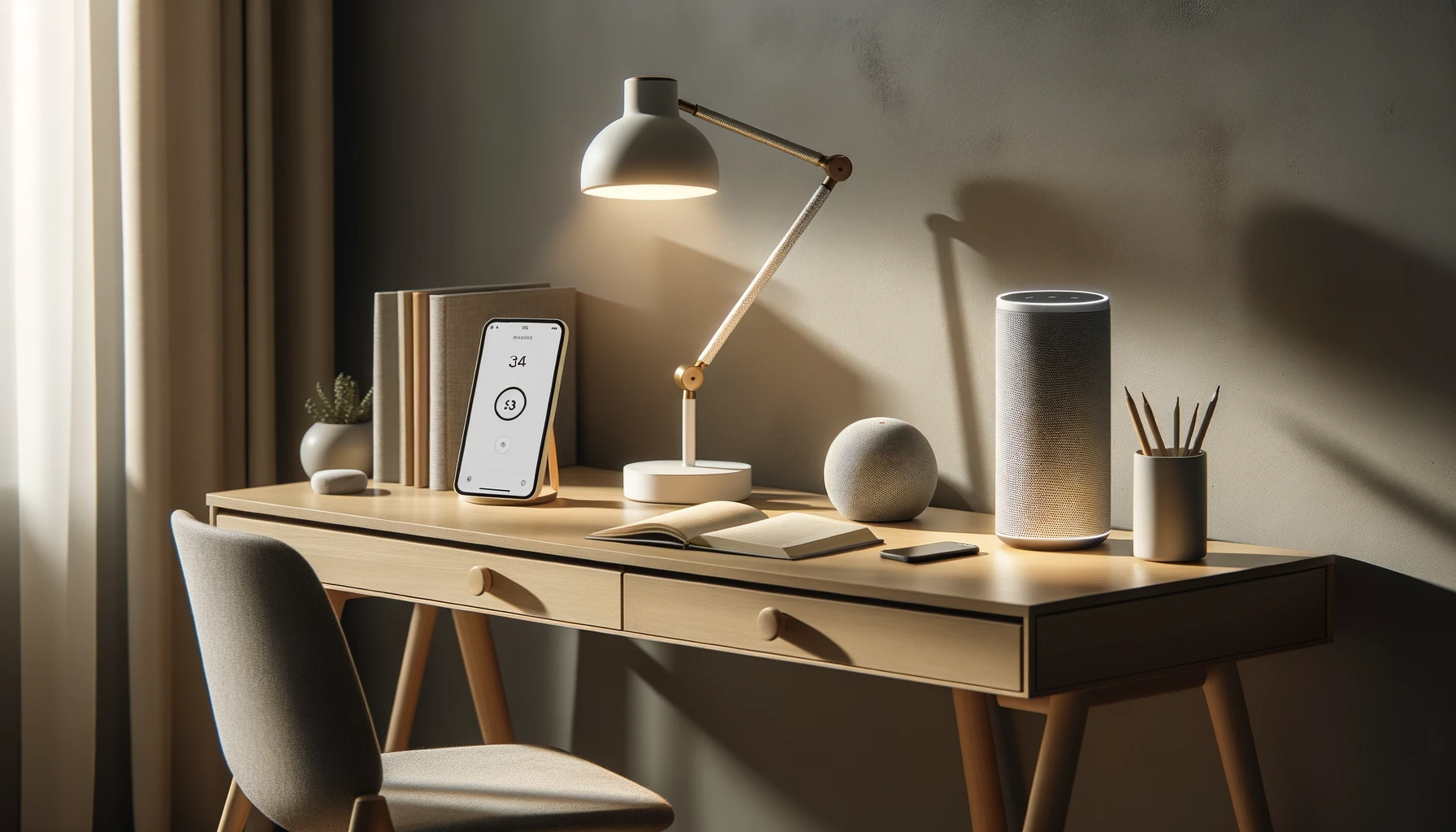The image depicts a cozy and neatly organized workspace featuring a narrow, light brown wooden desk with two drawers that have round wooden knobs. The desk, likely covered in veneer or lacquer, stands on long, slender legs that are angled for support. Positioned in front of the desk, slightly off to the side, is a simple chair with a gray cushioned seat and backrest, and light brown wooden legs.

On the desktop, to the left, there is a small white vase holding a green plant, next to a gray stone. Adjacent to these, four books stand upright in a row: two white, one orange, and one tan. Near the books rests a smartphone on a stand, displaying a countdown timer. Beside the phone, a white desk lamp shines a yellow light, casting a warm glow across the workspace.

Further right on the desk, an open book with white pages is placed, and behind it, there's a small gray spherical object. To the further right, a gray Amazon Alexa device sits beside a white cup filled with pencils. The desk is situated against a gray wall, with beige curtains visible on the side, creating a serene and functional work environment.